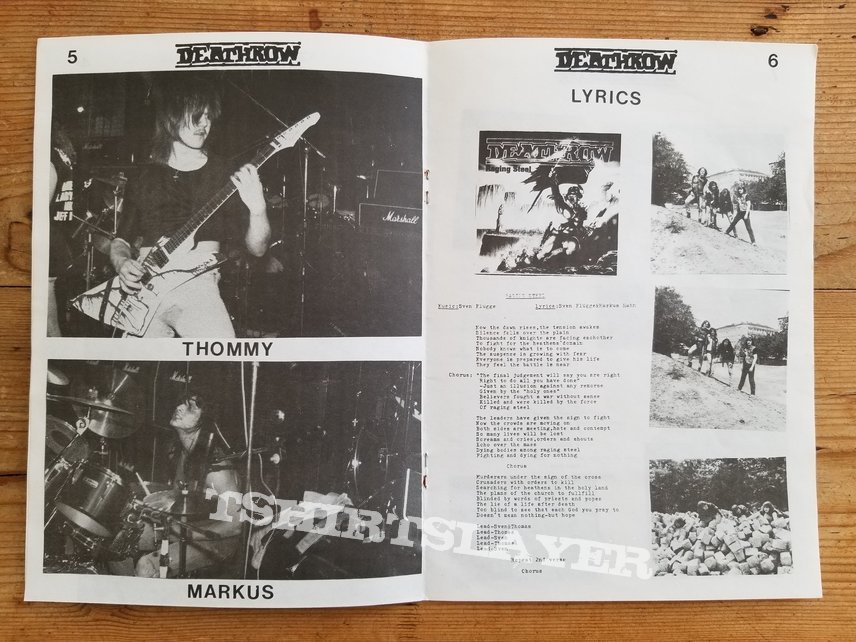The image showcases an open, vintage magazine or songbook, seemingly from the 60s or 70s, laid out on a brown, wooden table. The magazine is in decent condition and is predominantly black, white, and gray. In the center of the image is the open spread of the magazine, with the left page featuring black-and-white photographs of two band members: Tommy (T-H-O-M-M-Y) playing a guitar at the top and Marcus (M-A-R-K-U-S) playing the drums at the bottom. On the right page, there are four black-and-white photographs arranged in two rows — one photograph on the top left and three on the bottom right. Adjacent to these photos is a block of song lyrics that are printed in a small font, making them difficult to read. The lyrics page also features images of people standing on a hill. At the top of both pages, the handwritten all-cap style logo "Death Row" is prominently displayed. Additionally, the band name "Tommy and Marcus" is labeled on the left page. The numbers "5" and "6" appear at the top corners of the respective pages. Overlaying the bottom of the entire image is a watermarked brand name "T-Shirt Slayer" in a white western font. The setting suggests the magazine is being viewed on a desk or kitchen table, possibly in someone's home.